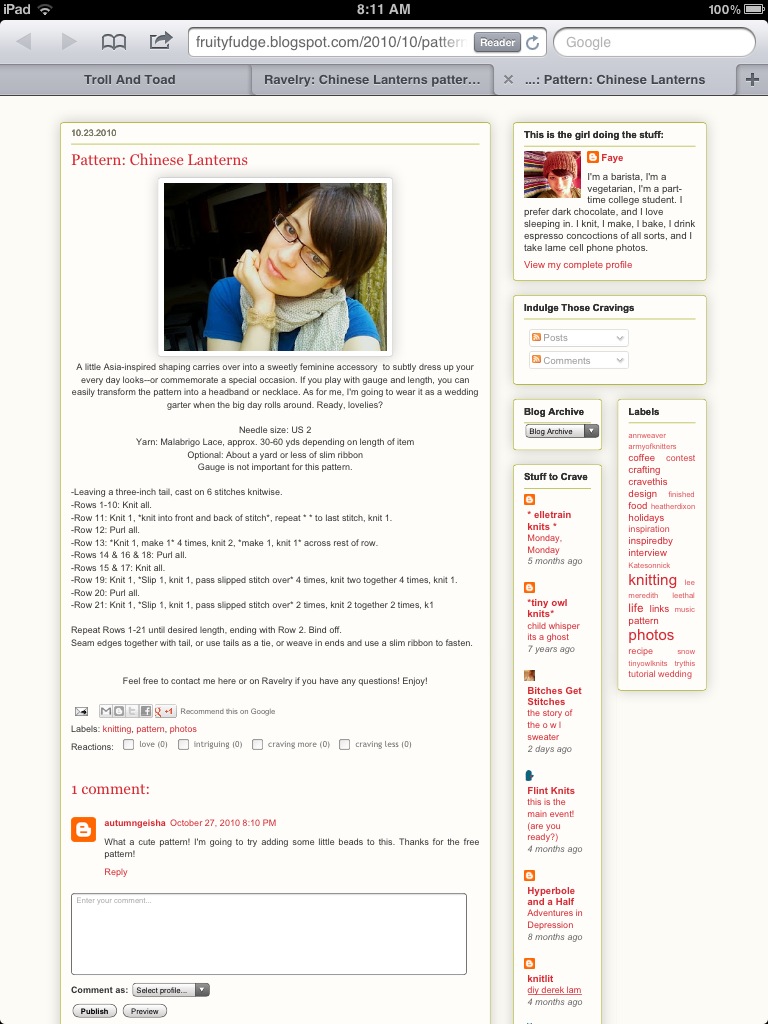The screenshot captures an iPad screen displaying a webpage in a browser, identifiable by the presence of the iPad's notification bar at the top. The left side of the bar reads "iPad," the center shows the time as 8:11 AM, and the right side indicates a fully charged battery at 100%. Below the notification bar, a browser window is open to the website fruityfudge.blogspot.com. Three tabs are visible, with the third tab titled "Pattern Chinese Lanterns," which is the active page displayed on the screen.

The title of the webpage reads "Pattern Chinese Lanterns" in red, followed by a close-up image of a woman with glasses, brown hair, and a blue shirt. The woman’s head is slightly tilted to the side. Beneath her picture is a detailed text description explaining how to make Chinese lanterns step-by-step. The background of the page is white, with the instructional text in black and some headings in red.

The bottom of the page features a comment section with one existing comment visible, along with a text box for additional comments. The page includes various elements like labels in red text, drop-down menus, and additional buttons, reinforcing the blog format of the website. The overall layout and features suggest that this is a blog post highlighting a pattern for creating Chinese lanterns.